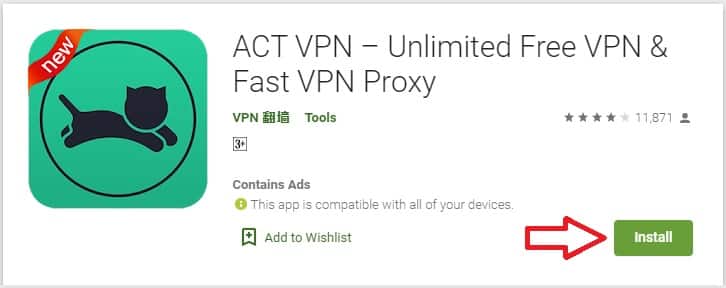The image appears to be a screenshot from a website, showing a small rectangular section rather than the full webpage. At the top, in gray font, the text "ACT VPN" is visible, followed by the description "Unlimited Free VPN and Fast VPN Proxy." Below this, the category "VPN Tools" is listed. On the left side of the image, the logo for the product is prominently displayed, featuring an aquamarine green square with rounded corners containing a black circle. Inside the circle is a minimalist, stylized black cat composed of simple black shapes, without detailed features such as eyes, yet clearly recognizable as a cat.

In the lower right-hand corner of the image, there is a rectangular, olive green button with the white text "Install." Alongside the button, a red-outlined arrow, filled with white, points towards the "Install" button, drawing attention to it.